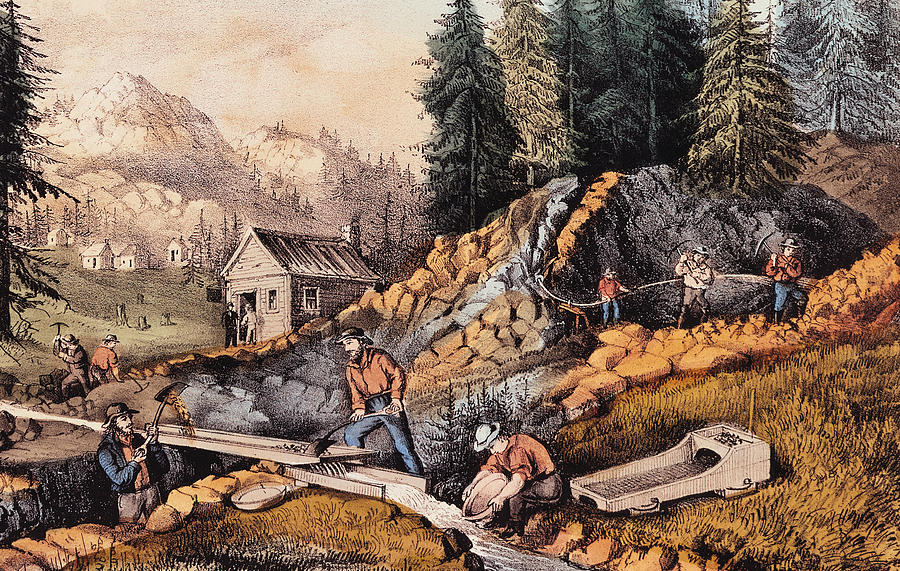This illustration, likely a drawing or painting, depicts a detailed mining operation set against a mountainous backdrop. The scene features workers on a mountainside, dressed in jeans and hats, using tools like shovels, pickaxes, and other hand tools. They are engaged in various activities, such as digging, scooping material onto a sluice, and sifting through bowls and sieves, likely in search of gold. To the left are a series of cabins or homes, including one larger building that appears to be the headquarters, with a figure outside in a suit suggesting he might be the boss. The background shows distant mountains and dotted houses, while the top right is adorned with pine trees. The palette is muted, with rustic oranges, greens, blues, and yellowy greens, contrasted by blacks and whites. There are approximately nine or ten figures engaged in the operation, some working on what seems to be water tracking or small tunnels. The overall scene captures the essence of a bustling, rustic gold-mining community.